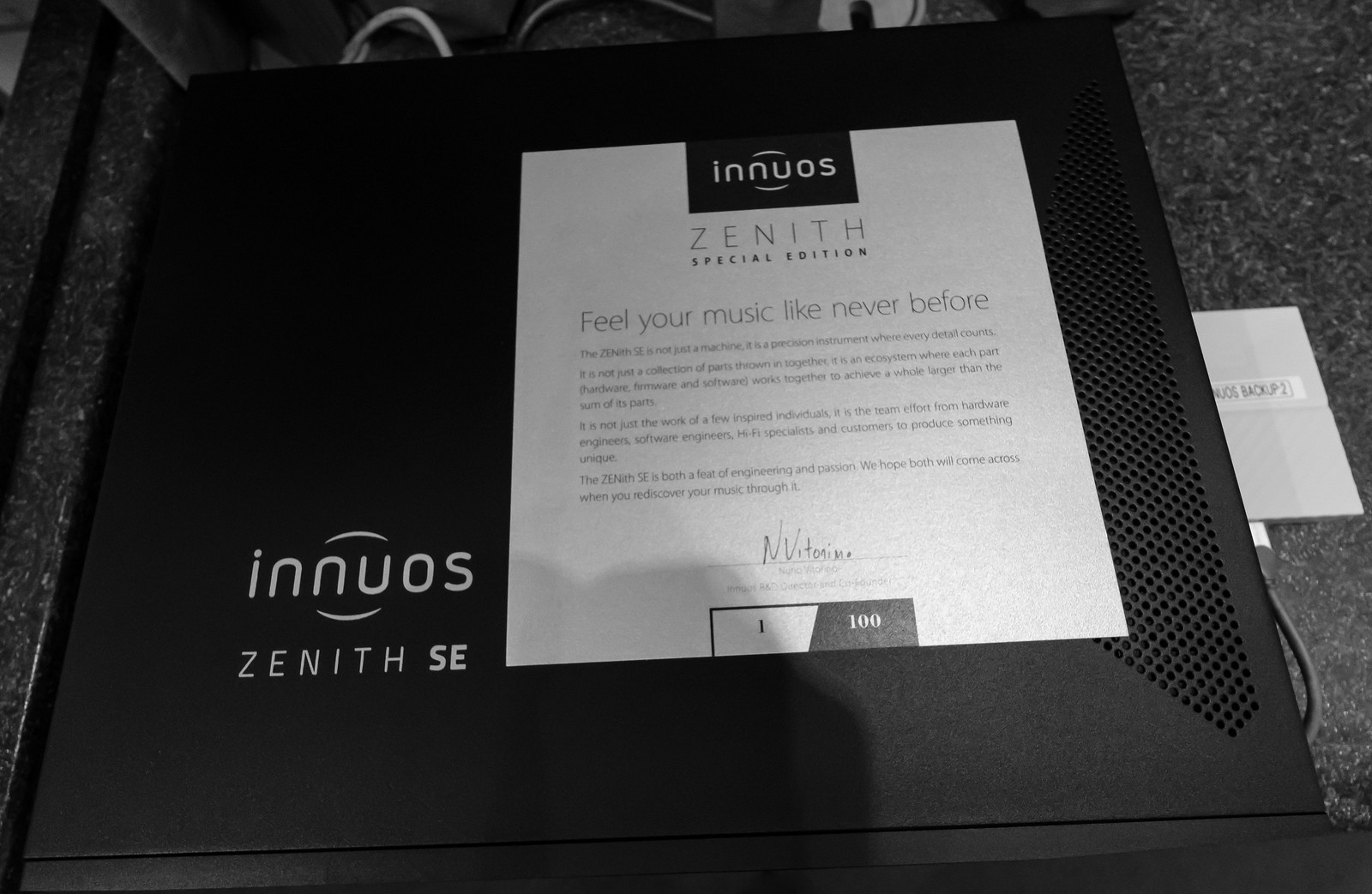The image depicts a sleek black device, resembling a hi-fi audio component or computer case, positioned against a background of gray foam and visible wiring. The device features a ventilated right side and is marked with a white logo on the bottom left that reads "Innuos Zenith SE," with the brand "Innuos" spelled I-N-N-U-O-S. Positioned on top of the device is a black and white paper, prominently displaying the same logo. The paper is inscribed with the text "Zenith Special Edition" followed by the tagline "Feel your music like never before." It emphasizes that the Zenith SE is not merely a machine but a precision instrument where every detail matters. The text expounds on how it is an ecosystem, where the synergy of hardware, firmware, and software creates a product greater than the sum of its parts. Furthermore, it highlights the collaborative effort of hardware engineers, software engineers, hi-fi specialists, and customers in bringing this unique device to life. The Zenith SE is portrayed as a culmination of engineering excellence and passion, designed to enhance the music-listening experience.